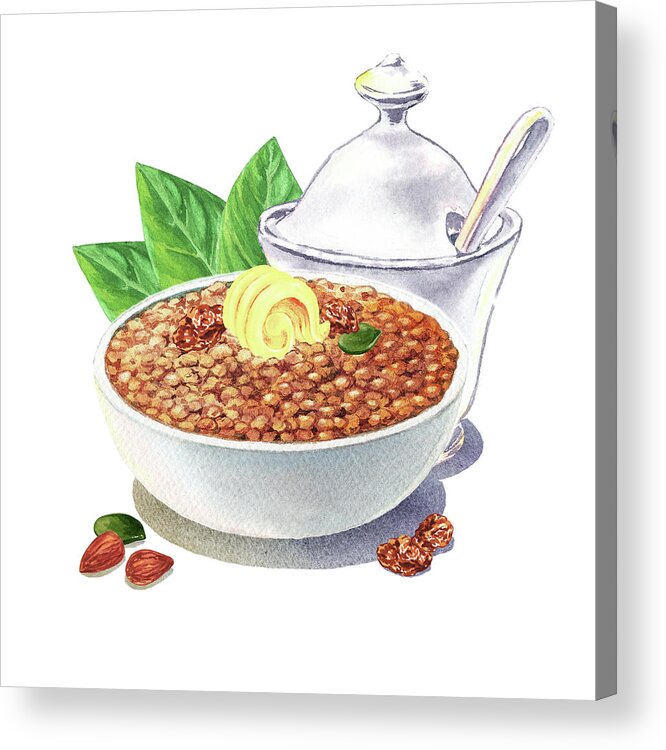This illustration on white paper portrays an artistically rendered, white bowl filled with various small, round fruits, likely cranberries, raisins, or prunes, accompanied by an elegant yellow swirl on top, possibly cheese or an edible decoration. Adjacent to the bowl is a typical sugar bowl with a lid, featuring a spoon protruding through its opening. In the background, three green leaves add a touch of nature to the composition. Shadows beneath the bowl and sugar bowl indicate the light source is above. On the left side of the bowl, several shelled brown nuts are visible, while on the right side, two additional nuts, a green leaf, and possibly some dates, raisins, or cranberries can be found. This meticulously detailed drawing captures the essence of a well-arranged serving set with an artistic flair.